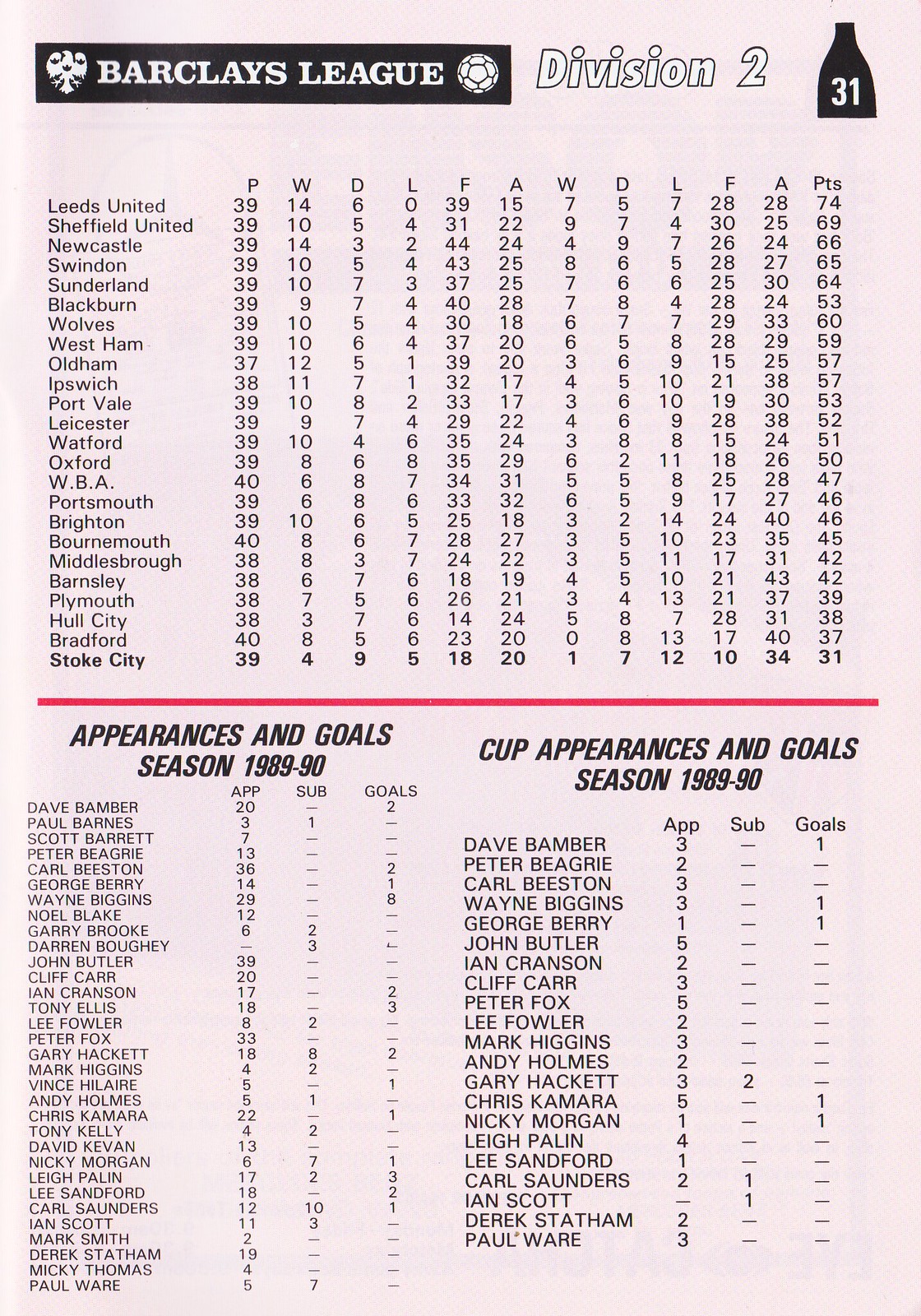This detailed poster features a stat sheet for the Barclays League Division II, highlighting the 1989-1990 season. It prominently displays a bottle-shaped black graphic with a white number 31, symbolizing the significance of Leeds United, which is listed first among the teams. The teams are arranged in multiple columns in descending order based on their win and loss records for the season. The list includes Leeds United, Sheffield United, Newcastle, Swindon, Sunderland, Blackburn, Wolves, West Ham, Oldham, Ipswich, Port Vale, Leicester, Watford, Oxford, WBA, Portsmouth, Brighton, Bournemouth, Middlesbrough, Barnsley, Plymouth, Hull City, Bradford, and Stoke City.

Additionally, the poster details individual appearances and goals, both for the season and for cup competitions in 1989-1990. The players named include Dave Bamber, Pete Bejry, Carl Beeston, Wayne Biggins, George Berry, John Butler, Ian Cranston, Cliff Carr, Peter Fox, Lee Fowler, Mark Higgins, Andy Holmes, Gary Hackett, Chris Kamara, Nikki Morgan, Lee Palin, Lee Sanford, Carl Sanders, Ian Scott, Derek Statham, and Paul Ware. The organized structure and detailed records make this poster a comprehensive reference for the 1989-1990 Division II season.